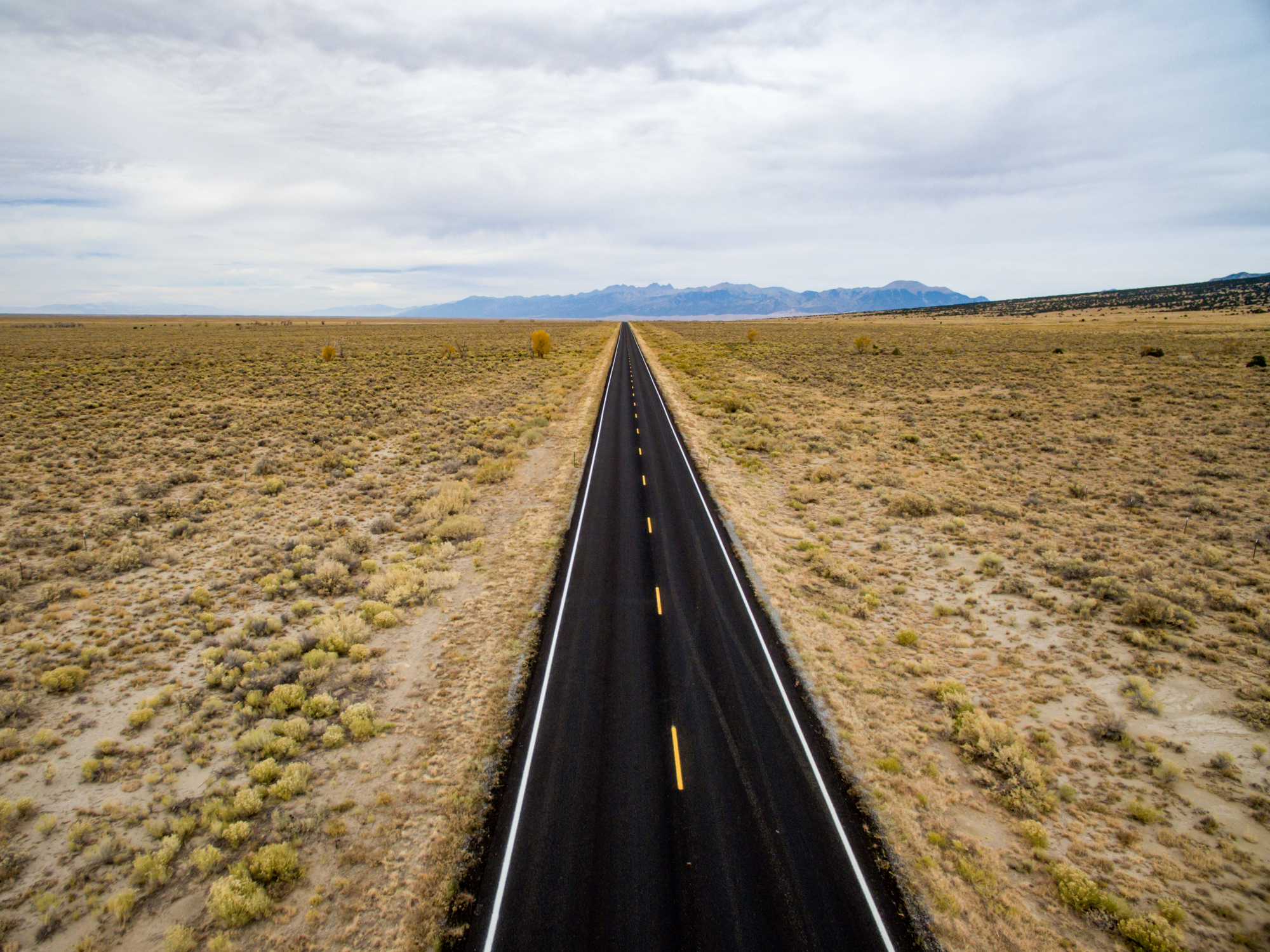The image captures a straight, freshly paved two-lane black road stretching into the horizon, marked by central yellow dashed lines and bordered by white shoulder lines. This road bisects a wide, flat expanse of scrubland, populated with low, sparse bushes in muted shades of yellow and brown, scattered over dirt. On the right side, a minor rise in the terrain is visible, while the distant background reveals more prominent hills or a mountain range, colored blue due to their remoteness. Dominating the upper portion of the image, the sky is largely cloudy, with shades varying from white to gray, and hints of blue peeking through predominantly on the left side. The overall scene conveys a daytime view of a desolate road cutting through a vast, dry plain.